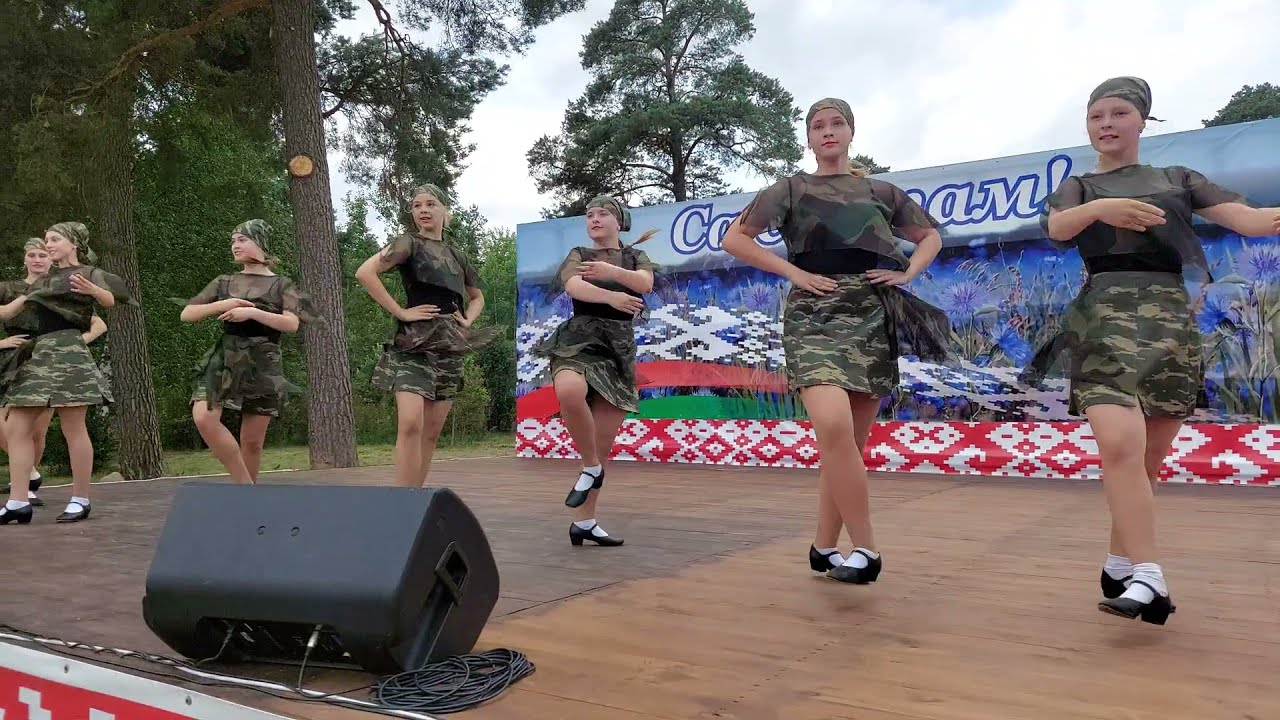The photograph depicts seven women dancing in unison on an outdoor wooden stage. They are dressed uniformly in camouflage attire, consisting of camouflage skirts, t-shirts adorned with black tank tops, and sheer camo-like fabrics. Each dancer complements her outfit with a camouflage scarf wrapped around her head, white ankle socks, and black Mary Jane shoes, which could be tap shoes. Positioned behind the women is a sizable blue sign, adorned with tribal graphic designs and possibly palm trees, contributing to the rustic, outdoor ambiance. Further enhancing the scenic backdrop, tall green trees and a bright blue sky with large, fluffy clouds are visible, situating the stage within a serene, wooded setting. In front of the dancers, a large black speaker can be seen, hinting at the musical accompaniment to their rhythmic performance that might resemble an Irish dance.